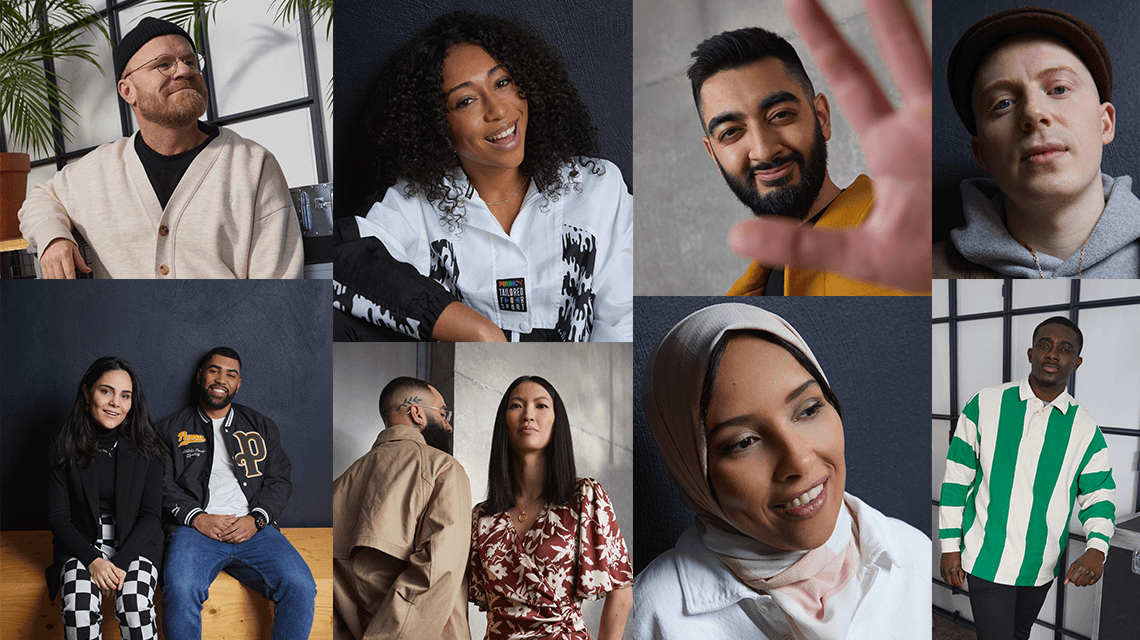The image is divided into eight distinct squares, each featuring a different individual. 

In the upper left corner, there is a man with red facial hair and small, circular glasses, dressed in a black t-shirt with a beige sweater over it. He is smiling slightly and gazing off into the distance. To his right, a woman with light brown skin and curly black hair is captured mid-laugh, wearing a black and white shirt. Next to her, a man with tanned skin, short black hair, and black facial hair is extending his hand in front of him. The person to the far right in this row has light white skin and a somber expression.

In the second row, two individuals are sitting side by side, each slightly smiling. The woman wears black and white checkered pants, while the man next to her is in jeans and a jacket with the letter 'P' on it. Following them, a man is seen from behind, showcasing his black facial hair and brown jacket. Beside him, a woman with straight black hair has a serious expression on her face. The next individual in this row is a woman in a headscarf, looking pensively into the distance. The final person is a man with dark skin and short brown hair, dressed in a green and white striped shirt.